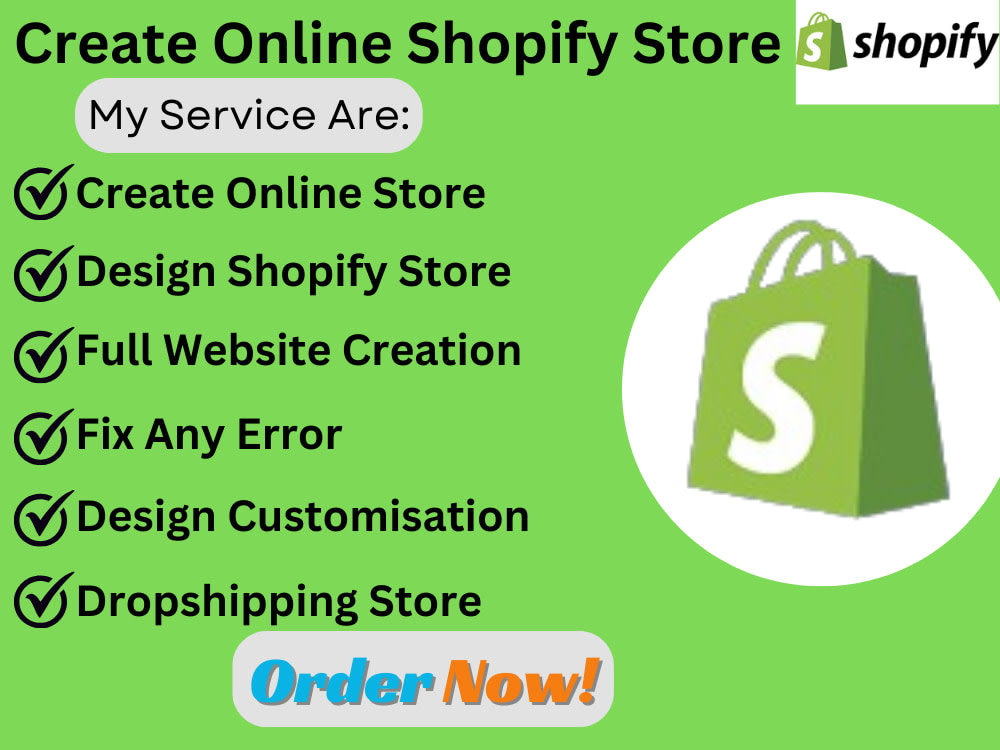The image is an illustration, predominantly in white and green, resembling a webpage promoting Shopify services. At the top right corner, it features the Shopify logo, depicted as a green shopping bag with an 'S' in white and "Shopify" written in black beside it. The primary text reads "Create Online Shopify Store," followed by listed services: "Create online store, design Shopify store, full website creation, fix any error, design customization, drop shipping store." At the bottom of the image, within a white oval shape, there's an "Order Now" button, with "Order" written in blue and "now" in orange with an exclamation point, aiming to prompt immediate action. The image uses clear, instructional language to guide users on creating a Shopify store and highlights various customization and troubleshooting services offered.